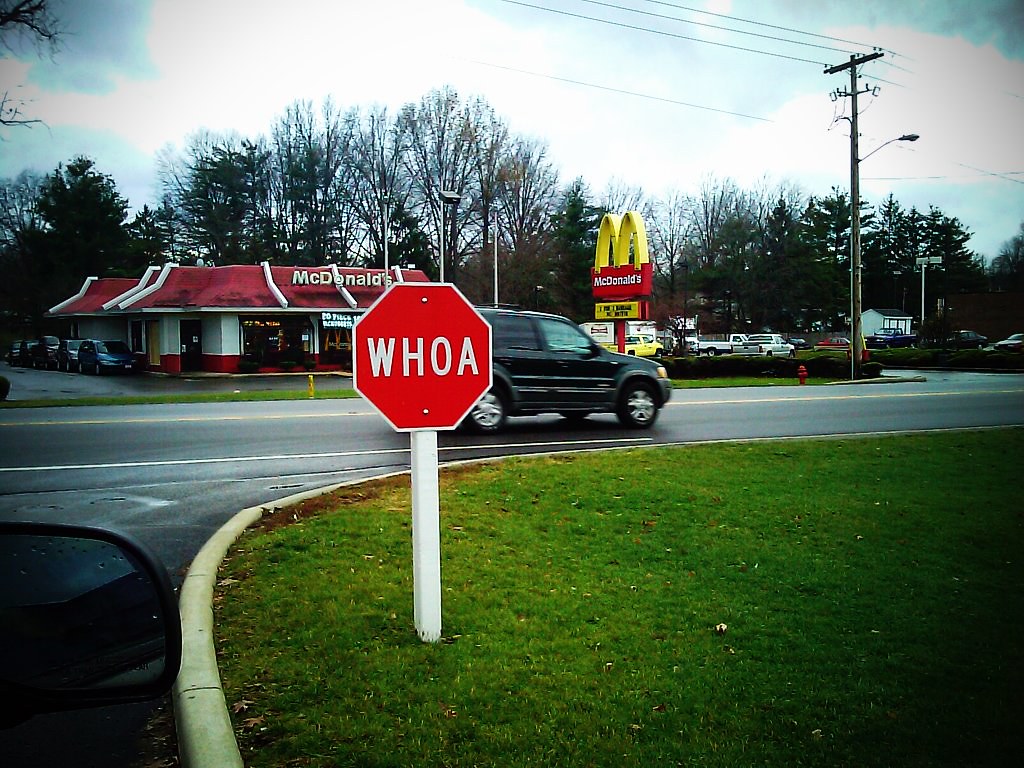The photograph captures an outdoor scene taken from a car window, likely from the passenger seat. Dominating the left foreground is the car’s side mirror, indicating the picture was taken mid-journey. At the bottom right, you can see the edge of the curb, a patch of dark green grass, and a white post that supports a distinctive red sign shaped like a stop sign, but instead of "STOP," it reads "WHOA" in white text. Ahead lies a road divided by a yellow center line, with a black SUV driving in front of the viewer’s car. Across the street stands an old-school McDonald’s with its iconic red roof adorned with white lines. The McDonald’s sign is prominently displayed in red and yellow. The scene is completed with additional cars in the McDonald’s parking lot and drive-thru, a backdrop of trees, a light pole with wires stretching across, and a sky transitioning through hues of light pink, blue, and white, suggestive of either dawn or dusk.